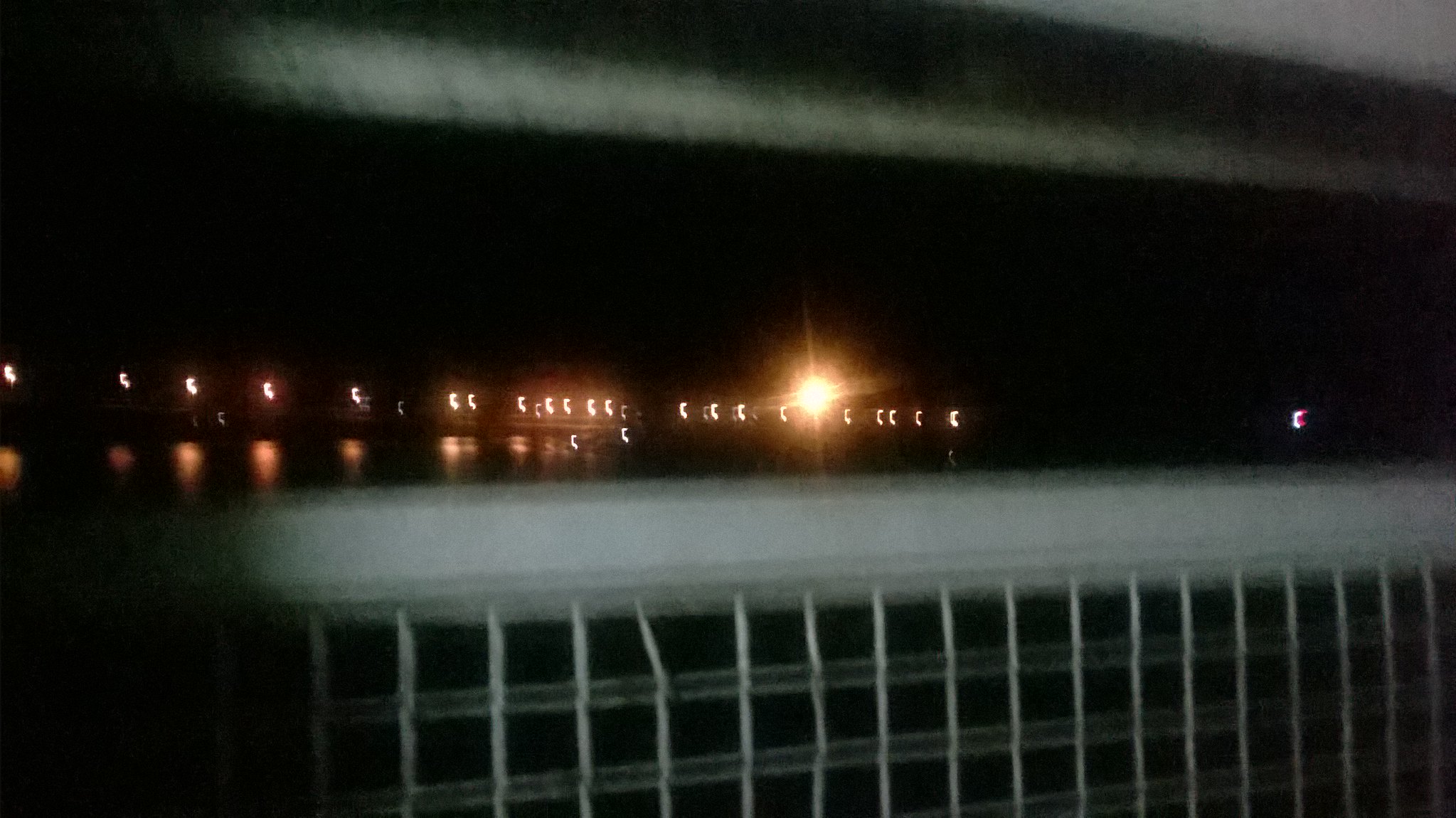This image is a horizontally-oriented, blurry nighttime color photograph, possibly taken from a moving car or while walking along a bridge. The lower portion of the image features a metal fence with a grid-like structure, extending from the bottom right corner to the left-hand side. The background is predominantly black, dotted with distant lights that appear streaked due to the camera’s movement. These lights reflect softly on the water below, creating a scattered pattern. Dominating the center is an intensely bright light, resembling a miniature glowing sun, adding a surreal element to the scene. The top of the image is framed by the upper section of the metal fence or a similar metal bar, stretching from the top right corner across to the upper left quadrant, mirroring the structure below.